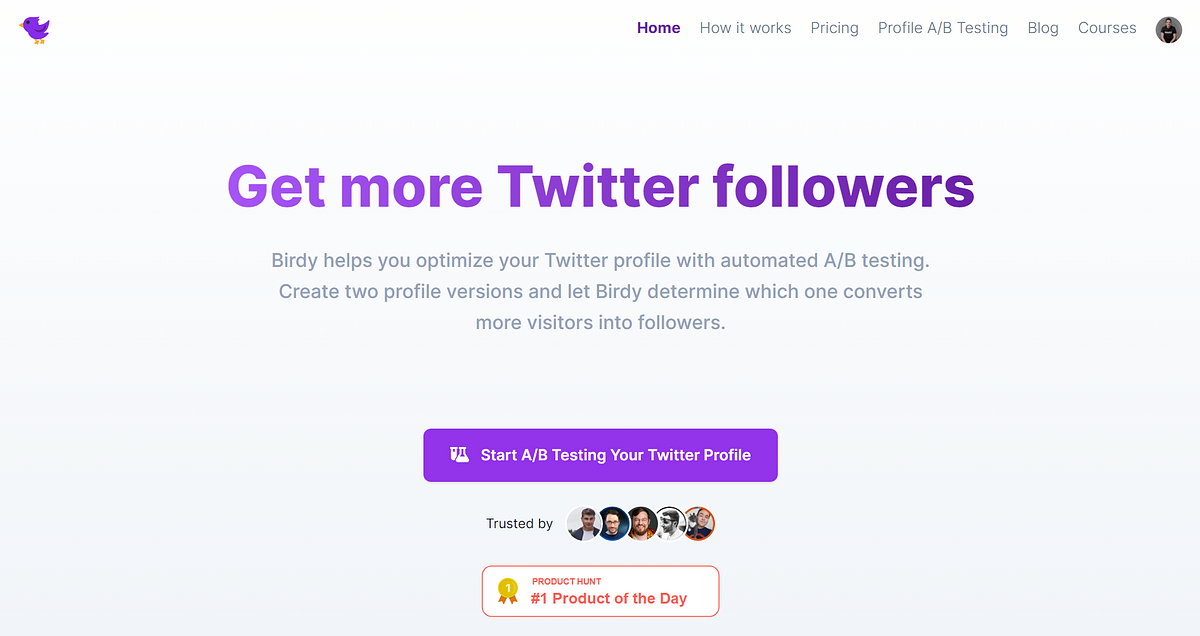Certainly! Here is a cleaned-up and detailed version of the original caption:

---

**Detailed Caption:**

The image features a webpage dedicated to explaining how to increase Twitter followers. The background is a subtle off-white or light gray color. In the top left corner, there's an illustration of a purple bird with an orange beak and small orange feet. Moving towards the right side of the page, a navigation bar includes bold text items such as "Home," followed by "How it Works," "Pricing," "Profile," "A-B Testing," "Blog," and "Courses." In the upper right corner, there is a circular photo of a man.

Dominating the middle of the page, in bold purple text, is the heading "Get More Twitter Followers." Just below, in dark gray or black text, the description reads: "Birdie helps you optimize your Twitter profile with automated A-B testing. Create two profile versions and let Birdie determine which one converts more visitors into followers."

Centered further down is a prominent purple rectangle with white text that reads, "Start A-B Testing Your Twitter Profile." Accompanying this text is a small icon resembling scientific vials, emphasizing the testing aspect. Additionally, the phrase "Trusted by" is listed with several circles featuring photos of various individuals.

At the bottom of the image, there's a white rectangle outlined with a red border, featuring a ribbon icon with the number one on it. It proudly declares, "Product Hunt, Number One Product of the Day."

---

This version provides a comprehensive and structured description suitable for understanding the content and layout of the webpage.